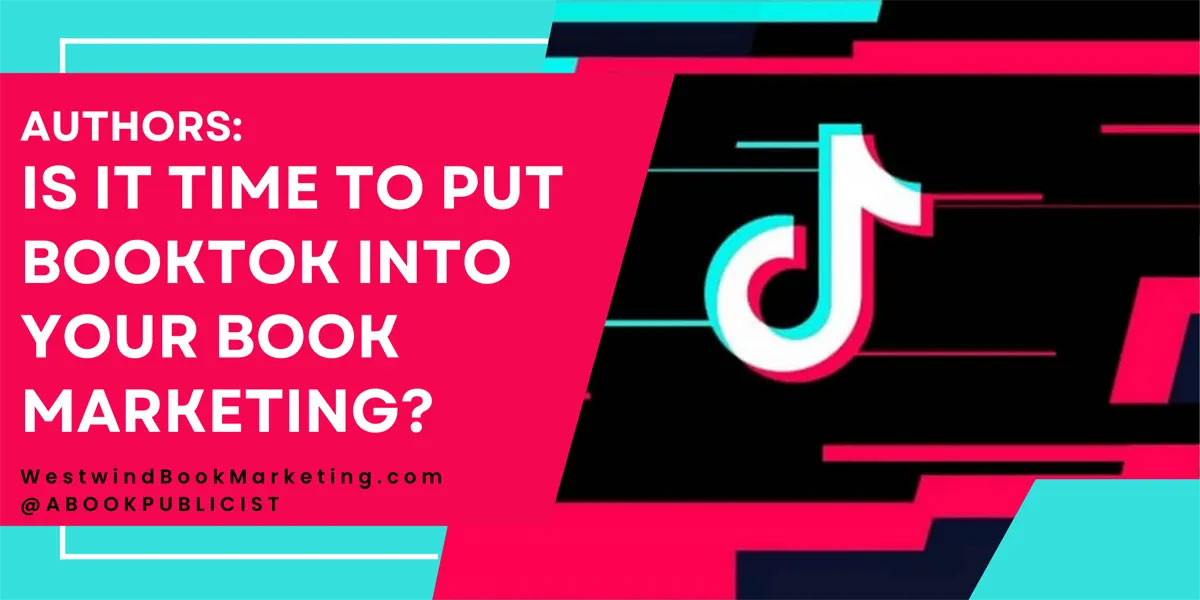The screenshot features an aqua background with an intricate design at its center. Prominently positioned in the top-left corner is a large red rectangle containing the following text in white, all capital letters: "AUTHORS:". Below this, in larger white capital letters, the text reads:

"IS IT TIME TO PUT
BOOK TALK INTO
YOUR BOOK
MARKETING?"

Two lines below this message, also centered, appears the text "westwindbookmarketing.com" in black. Adjacent to this, there is an "@" symbol followed by "ABOOKPUBLICIST" in black, all capital letters, without spaces.

Inside the red rectangle, towards the bottom right, a black rectangle is embedded. This black rectangle contains the TikTok logo on its left side. The left part of the TikTok logo may depict a stylized lowercase "n" in red, though it is somewhat ambiguous. Within this black rectangle, several horizontal aqua and red lines are visible, adding complexity to the design. The black rectangle extends downward into a small black square at its bottom center. At the lower right of this black rectangle is another red rectangle, which also features a small black square on its top right.

Above the central red rectangle, a white line starts from the center left, continues downward, disappears behind the red rectangle, reappears at the bottom, and extends to the right until it meets the edge of the rectangle again, creating a circuitous path.